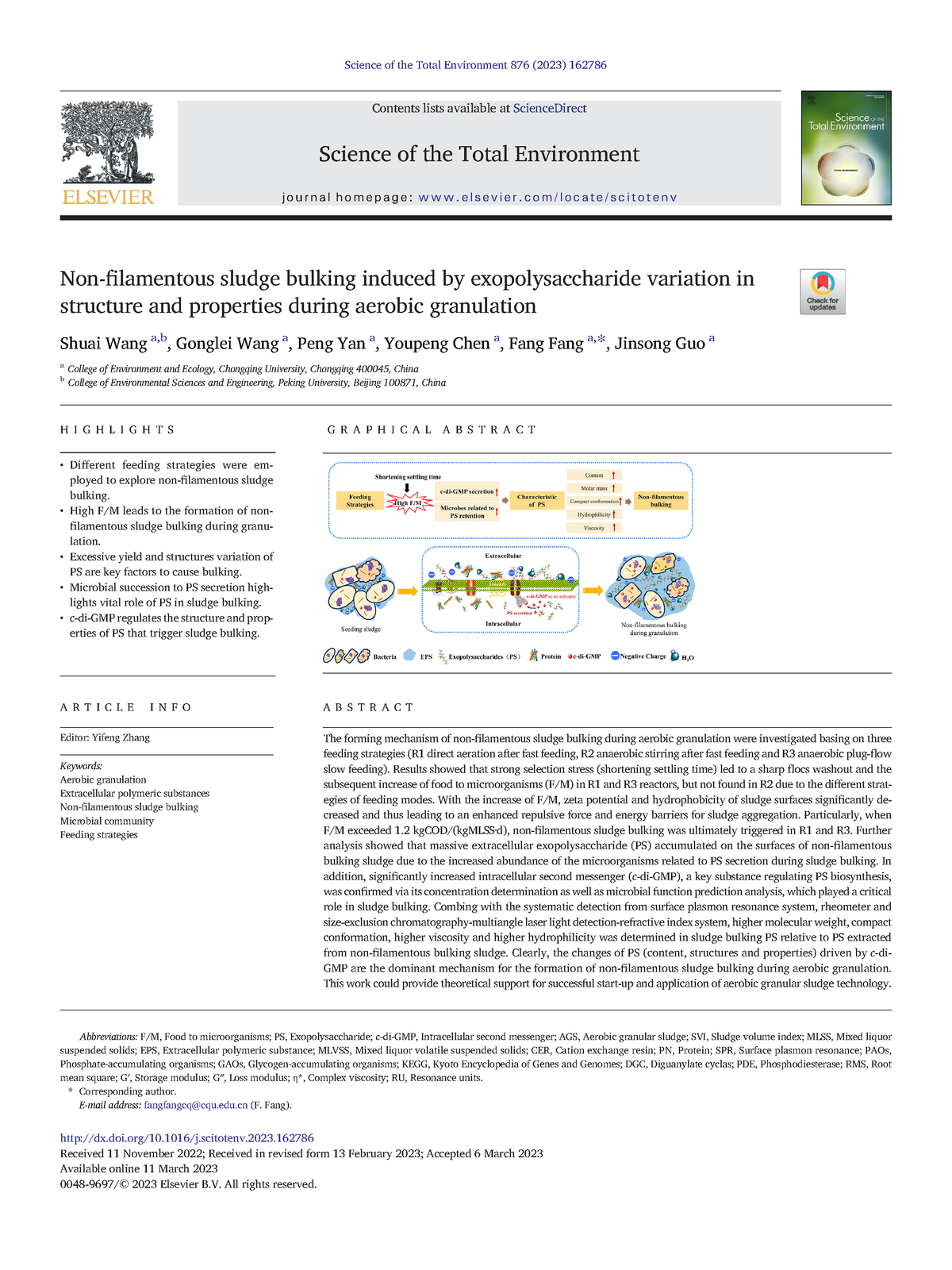In this detailed photographic image, we observe a webpage from a scientific journal. In the upper left-hand corner, a black and white graphic image of a tree is displayed alongside the text "Elsevier" in yellow writing. A gray banner spans the top of the page, featuring the title "Science of The Total Environment."

Beneath this banner, a blue hyperlink labeled "Journal Home Page" is visible, leading to additional journal resources. To the right side of the image is what appears to be a journal cover, characterized by a gradient of green, yellow, and white colors. The title on this cover reads: "Non-filamentous Sludge Bulking Induced by Exopolysaccharide Variation in Structure and Properties During Aerobic Granulation."

The authors of this featured paper are listed at the top in small text, including names such as Shui Wang, Guang Lei Wang, Peng Wang, Peng Yan, Yu Peng Chen, Feng Feng, and Jinsang Guo.

Further details on the page include sections titled "Highlights," "Graphical Abstract," "Article Information," and "Abstract," suggesting a standard research article layout typical for scientific publications.